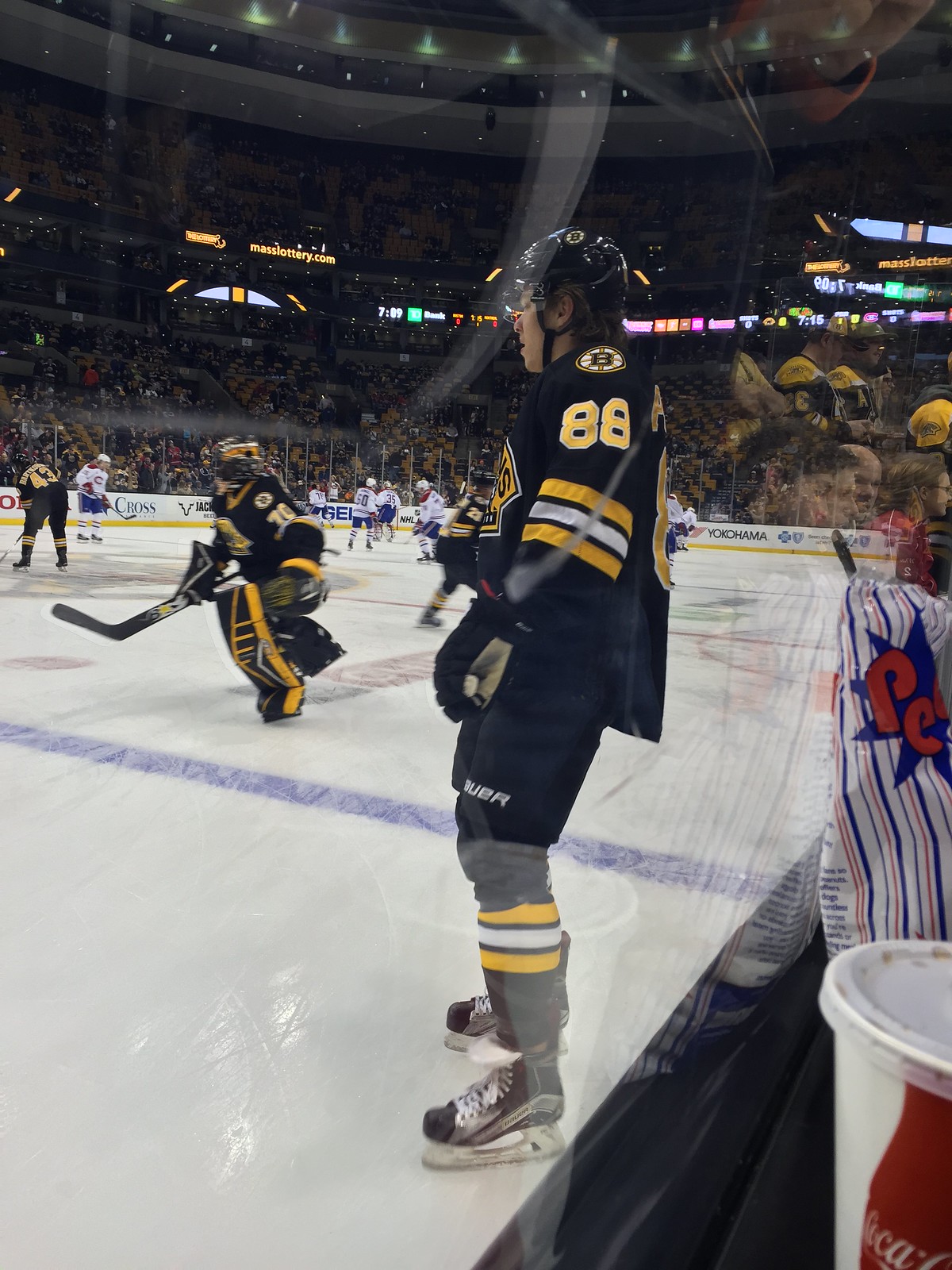This photo captures an intense moment at a National Hockey League game from the perspective of a fan seated behind the glass at the bottom of the stadium. The central focus is on a Boston Bruins player, jersey number 88, who is standing prominently near the stands. The player is dressed in a black jersey featuring yellow, white, yellow stripes on the sleeves, with matching socks and a black helmet. The number 88 is clearly visible on his left sleeve. In the background, the Bruins' goalie, fully equipped with protective gear, maintains his position against the opposing team, possibly the Calgary Flames given the color hints, though it's not entirely clear.

To the right of the player number 88, there is a white and red Coca-Cola cup sitting on the glass, suggesting the presence of a fan nearby. Behind the cup, a bag of candy with a red and blue design adds a splash of color. The vibrant scene includes various digital signs, advertisements, and neon lights illuminating the upper levels of the packed stadium. Spectators fill the seats, enhancing the atmosphere with a lively buzz, while ticker boards and clocks provide crucial game information. Despite the glare and reflections on the glass, the excitement and energy of the game are unmistakably captured in this detailed snapshot.